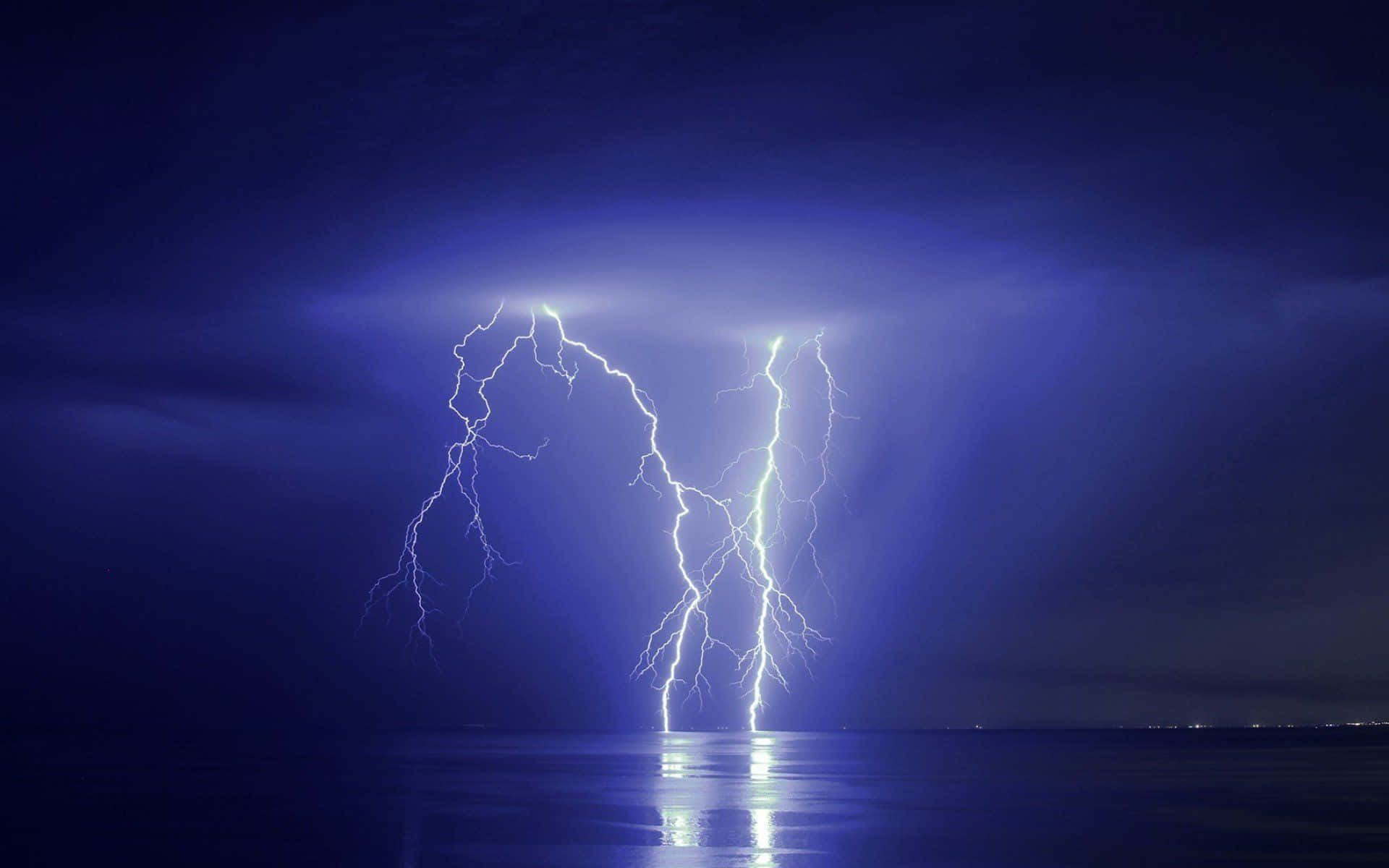This captivating nighttime photograph captures the raw power of nature, featuring two prominent lightning bolts striking over a vast body of water, possibly an ocean or large lake. The sky, an extraordinary gradient of purples, begins as a deep, dark purple at the top of the image and transitions into a fluorescent, lighter purple closer to the lightning bolts. This ombre effect beautifully highlights the electric spectacle unfolding mid-sky. The image's rich hues are reflected on the water below, adding depth to the scene. The lightning bolts, including subsidiary branches, form almost an H shape against the dark evening sky, vividly illuminating the atmosphere. To the right-hand side of this rectangular photograph, which is about twice as long as it is high, small electric lights on the distant shoreline suggest the presence of a city experiencing the storm. The combination of natural and artificial light, the stunning color palette, and the dramatic lightning bolts make this image a mesmerizing portrayal of a stormy night.